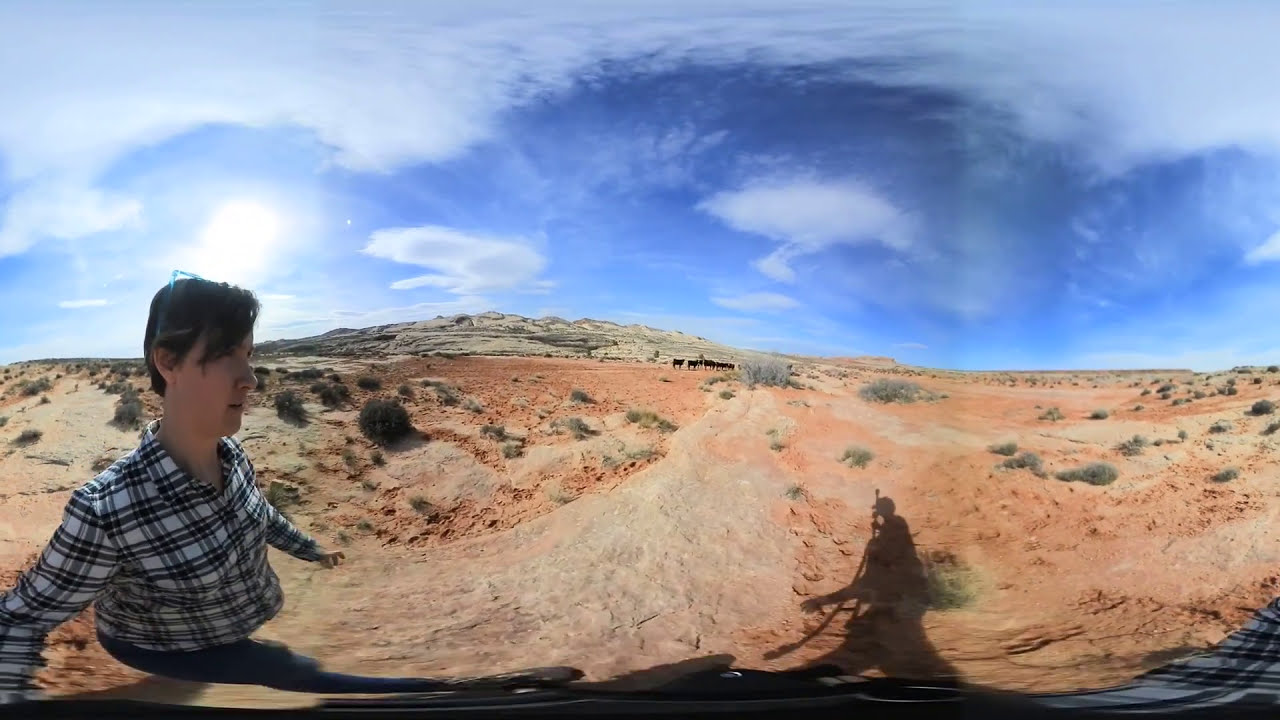In this distorted fisheye lens photograph of a desert scene, the foreground is dominated by a woman with short brown hair and glasses atop her head, clad in a black and white plaid shirt and blue jeans. She stands on the left side of the image, her leg stretched out far in front of her due to the lens's effect, while she gazes towards the right. The arid ground beneath her is light reddish-brown, interspersed with sparse desert vegetation, including dark green and yellow grasses, weeds, and possibly tumbleweeds. On the right side of the photo, the shadow of another individual is visible, depicted in a dramatic stance walking towards the left. This shadow, striking and somewhat menacing, shows one hand outstretched and another holding a stick above the head that aligns with the person's foot. In the distance, a herd of black cattle grazes near rocky, gray mountains under a blue sky largely blanketed by gray and white clouds, with a bright sun attempting to pierce through directly above the shadowed figure.